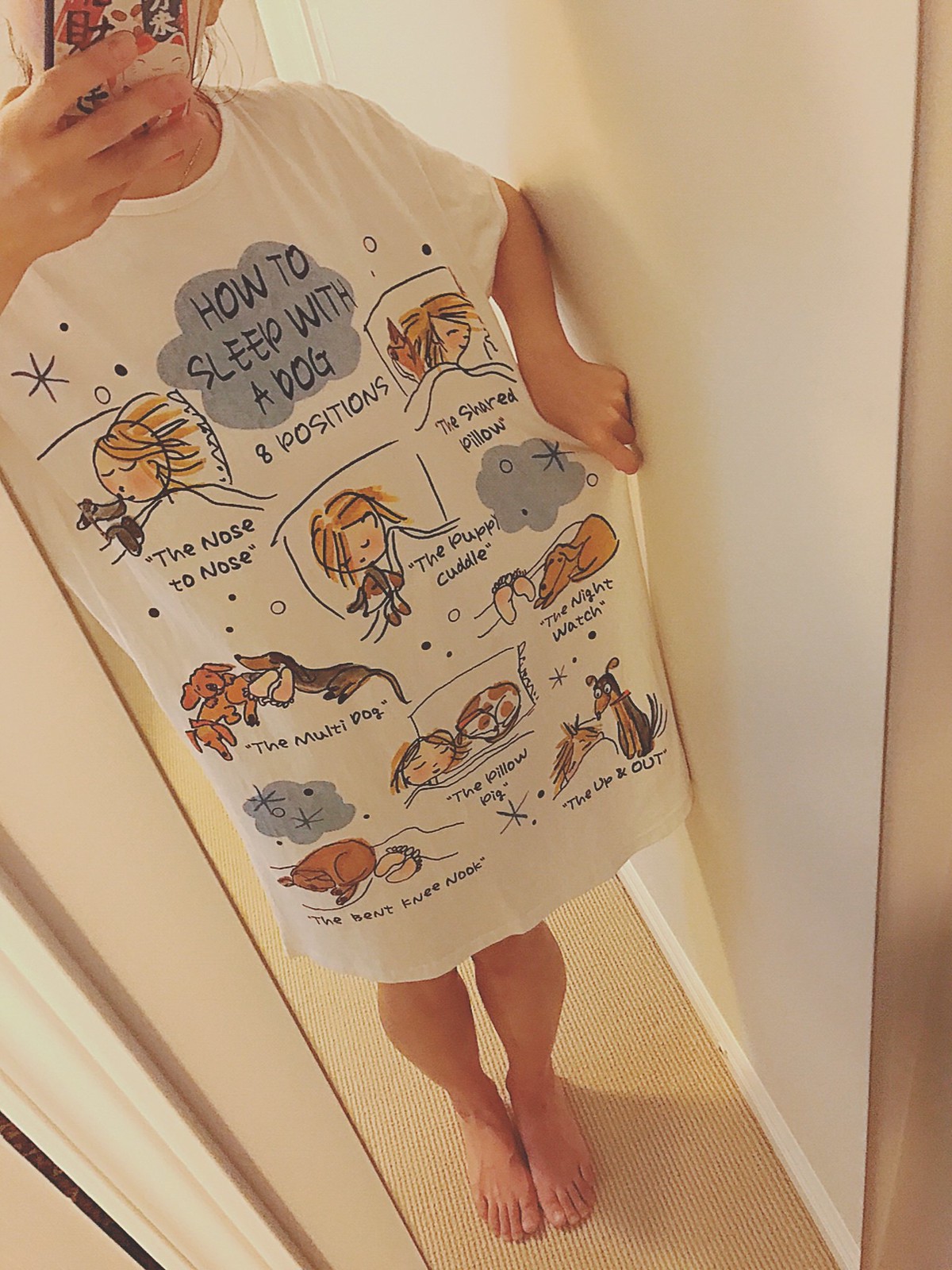The indoor color photograph features a young woman with light brown hair, wearing a white long shirt that reaches her knees, barefoot and standing on a textured, light tan carpet. She is holding a camera with a red and black design in her right hand, capturing a selfie in a full-length, frameless mirror mounted on a pure white wall. The focus of the image is her shirt, which she is pulling taut with her left hand to better display its design. The shirt humorously illustrates "How to Sleep with a Dog: Eight Positions" in simplistic, sketched cartoons. The drawing depicts a girl and various brown dogs in different sleeping positions such as the nose-to-nose, the shared pillow, the multi-dog, and others. The background of the shirt includes cloud and star patterns. The phone case features a Japanese lucky cat with Japanese writing, adding a unique detail to the overall scene.